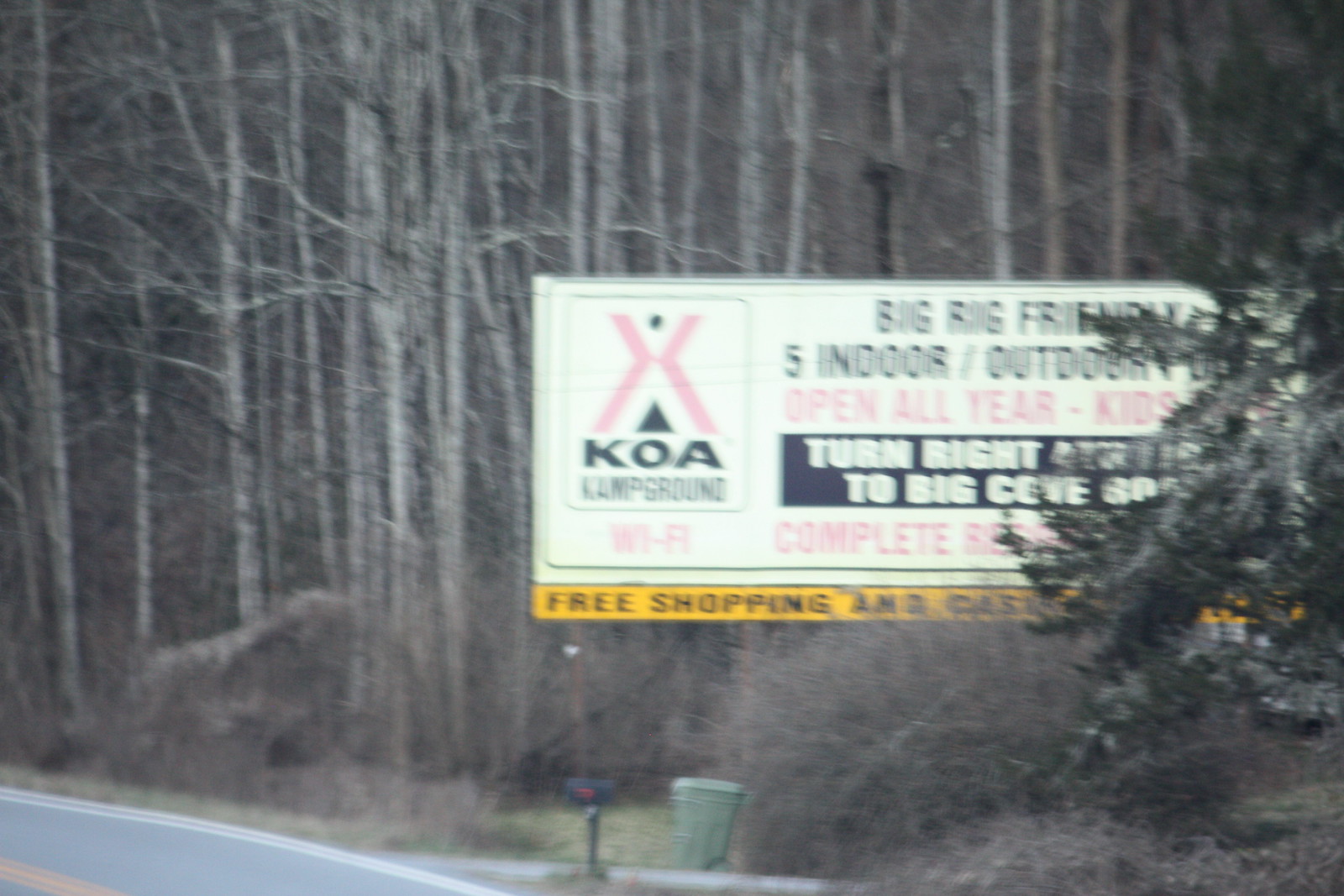This image appears to be an older photograph or perhaps one taken with a low-quality camera, depicting a forested area intersected by a road. The bottom-left corner of the image is slightly cut off, but it clearly shows a variety of trees, most of which are bare, except for one evergreen tree situated in the foreground on the right. Surrounding the road, there are smaller bushes and scrub. A driveway with a mailbox and a trash can can also be seen in the image. Above this driveway is a prominent sign that reads "Big Rig Friendly, 5 Indoor Outdoor All Year Kids Campground," showcasing the KOA (Kampgrounds of America) insignia. The scene evokes a rustic, somewhat desolate atmosphere, punctuated by the welcoming sign for the year-round campground.